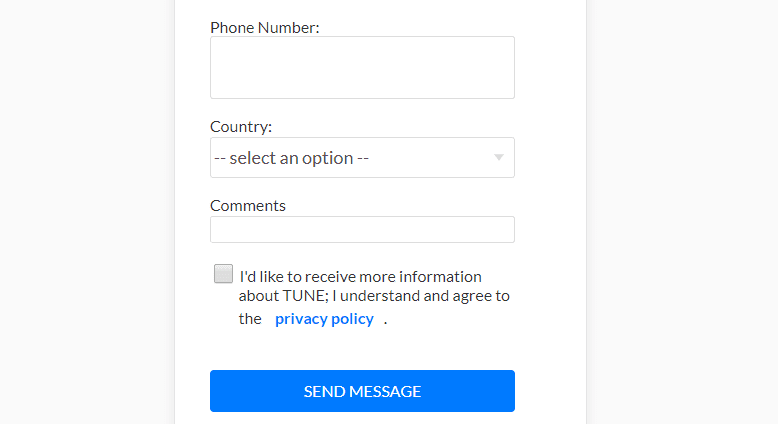The image is a zoomed-in screenshot of an online form set against an uninteresting grey background. Dominating the center of the image is a prominently white text box containing several interactive fields. At the top, there is a section labeled “Phone Number” with a corresponding white input box for users to enter their phone number. Below this, another section labeled "Country" features a dropdown menu indicated by the placeholder text "Select an option" and a grey downward arrow, allowing users to choose their country from a list. 

Further down, a narrower field is designated for "Comments," providing space for users to input their thoughts or inquiries. Directly beneath this is an unchecked grey checkbox, accompanied by the sentence in black text, "I'd like to receive more information about Tune, I understand and agree to the," with "privacy policy" highlighted in blue, indicating a clickable link to the policy details. To conclude the form, a blue “Send Message” button with white text is prominently displayed at the bottom.

The layout is simple and utilitarian, focusing on the interactive elements of the form without any additional decoration or background detail. Users can interact with the phone number and comments fields, select their country from the dropdown menu, check the box to receive more information, and ultimately, click the “Send Message” button to submit the form.